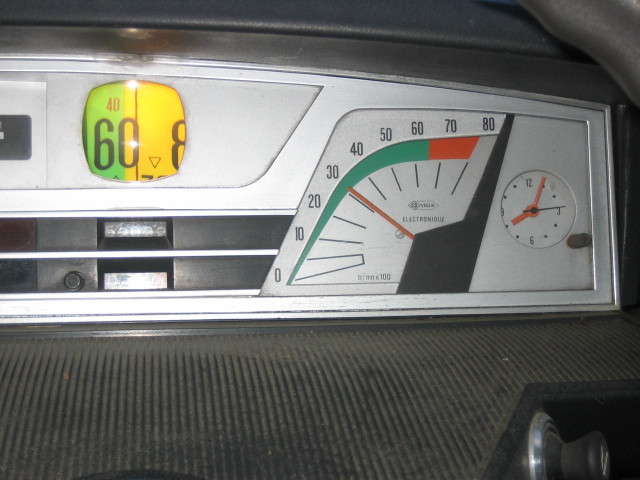The image is a color photograph capturing the detailed interior dashboard of a vehicle. The primary focus is the speedometer, positioned prominently on the right-hand side. Unlike traditional circular speedometers, this one features a red needle moving across a 90-degree curved arc. Starting from a narrow baseline at the bottom left, the arc gradually widens as it ascends diagonally, curving slightly past the horizontal mark and ending at the 80 mark. The gauge is divided into sections, with a green area transitioning into red at 60. The speedometer displays numbers in 10-unit increments from 0 to 80, with the needle currently positioned just above the 30 mark.

To the right of the speedometer is a clock with a distinctive face. The red hour and minute hands indicate the time as 8:05, while a black second hand sits just above the 3, pointing at the 14-second mark. The clock adds a classical touch to the modern dashboard setup.

In the bottom right corner of the image, a cigarette lighter is visible. It features a grey, graspable protrusion with a white sketch of a cigarette and smoke, seen from a side-on angle. This placement provides a nostalgic nod to older vehicle designs.

To the left of the image, another illuminated readout can be seen through a translucent plastic or glass covering. This secondary display is divided into green and yellow sections, with a vertical separation passing through the zero. The numbers '60' in black and '40' above it in smaller font are clearly visible within this display, contributing to the comprehensive data available to the driver. 

This meticulously detailed interior reflects a blend of functionality and aesthetic, catering to both traditional and modern automotive sensibilities.